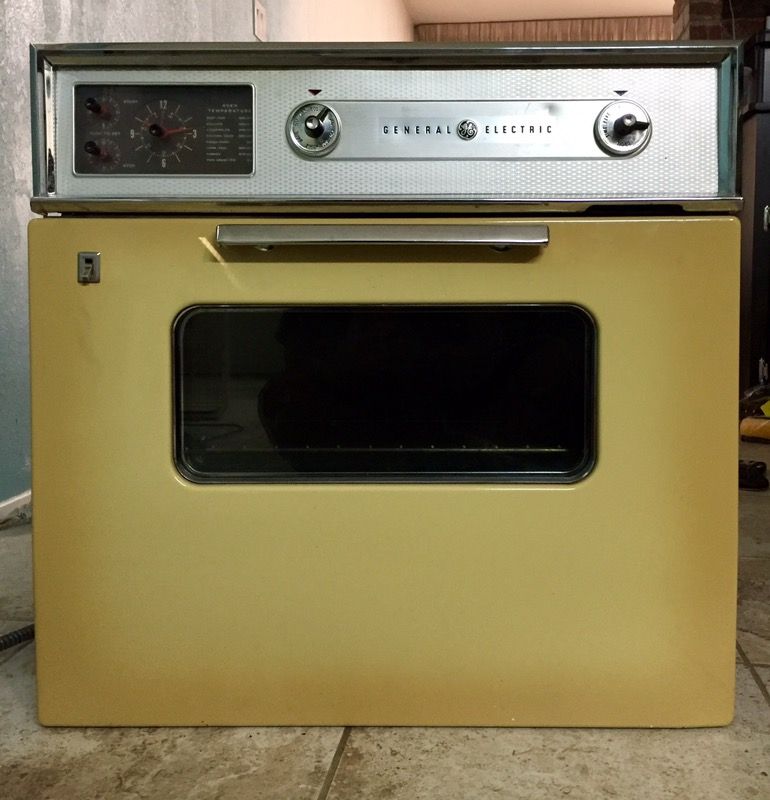This photograph showcases a vintage General Electric oven, likely from the 1960s or 70s, noted for its mustard yellow door, a popular kitchen color from that era. The top of the oven is metallic silver with chrome accents, and prominently features the "General Electric" branding, complete with the GE symbol between the words. Flanked by two silver control knobs, one on each side of the logo, the design suggests these may be used to manage the oven burners. On the left side, there's a small glass window displaying analog instruments, possibly for temperature and other settings, with additional small knobs for precise control. The oven door, finished in yellow, features a silver pull-down handle and includes a window revealing a metal baking rack inside. Adjacent to the door, a switch resembling a light switch is likely intended to illuminate the oven's interior. The oven sits on a tiled floor, against a backdrop of wall paneling and a soffit, indicating it has been recently removed from its original kitchen setting.